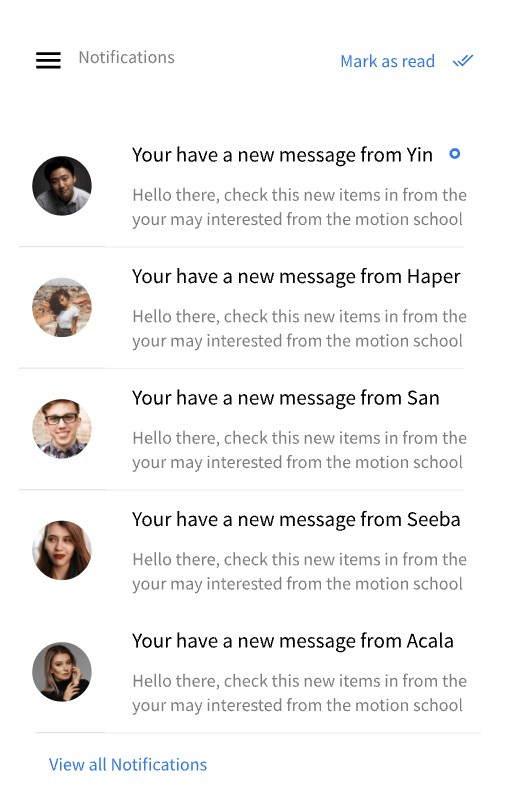The image depicts a notifications interface designed to display messages from various contacts. In the top left corner, there are three horizontal lines, commonly representing a menu button. To the right of this icon, the heading "Notifications" is prominently displayed. Adjacent to it, on the top right, there is a "Mark as Read" option in blue, accompanied by a double check mark icon.

Below the header, the interface lists several messages, each accompanied by a small profile picture of the sender. The first message is from an Asian man in a white shirt, identified as Yen. It reads, "Hello there, check this new items..." providing a brief preview of his message. The second message is from a woman named Happer, with a similar preview format. Following Happer, messages from three more contacts—Sam, Siva, and Akala—are displayed in the same manner.

At the bottom of the notification list, a blue hyperlink labeled "View All Notifications" invites users to access a comprehensive list of their notifications. The use of the color blue on this hyperlink suggests it is clickable, likely leading to a detailed view of all received messages beyond the five displayed in this sample. This interface effectively summarizes incoming messages by showing the sender's name, profile picture, and a snippet of the message to give users a quick glance at their recent notifications.